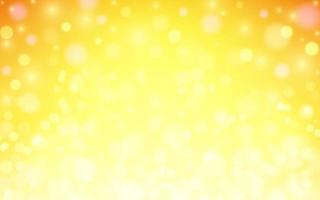A vibrant yellow background, suitable for a cellphone, tablet, or computer desktop, dominates the image. The rectangle of bright yellow gradually transitions into a rich gold hue at the top corners, adding depth and contrast. Scattered across the top and corners of the background are clusters of blurry pink and white dots, creating a soft, out-of-focus pattern that adds texture without distracting from the overall simplicity. The blend of bright yellow and gold, coupled with the delicate, misty dots, makes for a visually appealing and versatile background.